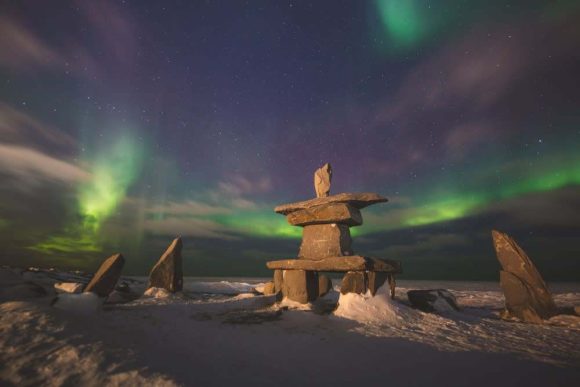The image depicts a stunning nighttime scene of the Northern Lights in Canada, with vibrant purples and greens dancing across a cloudy sky. The snow-covered landscape is dotted with primitive-looking stone sculptures, reminiscent of ancient monoliths. The focal point is a main stone structure composed of seven stacked layers, including upright rocks supporting flat, rectangular stones, culminating in a unique rock sculpture adorned with an X. To the right and left of the central monument, smaller, triangular stone formations jut out at angles from the snow, adding depth to the scene. The boulders are light brown and dark gray, contrasting vividly against the white snow and the colorful aurora borealis. The photograph, likely taken with a digital camera, captures a serene and mesmerizing natural spectacle, highlighted by faint, bright white stars scattered across the sky.